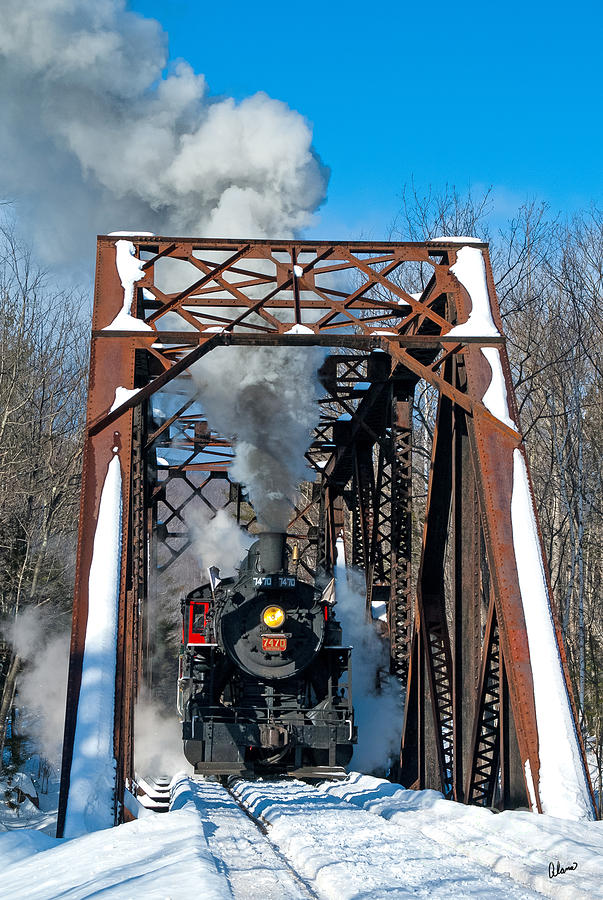The image captures a striking scene of a vintage black steam locomotive, identified by the number 7470 displayed prominently in white text on a red background beneath its yellow circular headlight. The train, billowing thick clouds of smoke from its smokestack and steam from underneath, chugs along snowy tracks laid across a rusted metal bridge. The bridge, constructed from large steel beams and cross posts, arches slightly before leveling out, and lacks any roofing or side walls apart from the steel supports. Snow blankets the entire scene, including the tracks and the bridge, while barren trees line both sides of the structure. The photo is taken from a perspective that suggests the viewer is standing close to the tracks, almost at eye level with the train, capturing the imposing presence of the locomotive as it seems to surge forward, kicking up snow in its path.